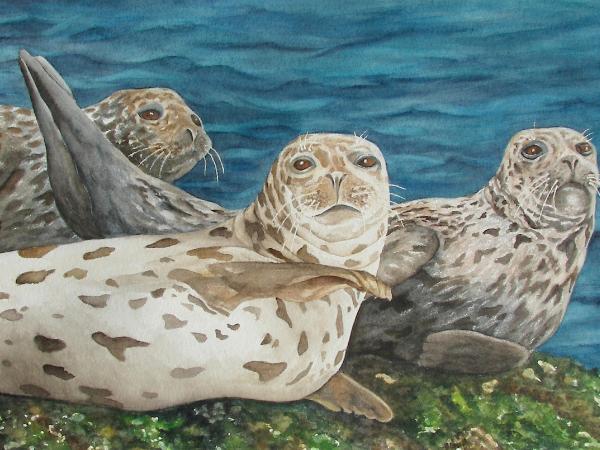This painting vividly captures three sea lions lounging on a green, flecked rock in front of a deep blue ocean. The distinctively colored sea lions are positioned in a staggered, overlapping arrangement, each appearing to look directly at the viewer. The foremost sea lion, appearing predominantly white with a few brown spots, strikes a relaxed pose, leaning back with a flipper raised. This "Dalmatian-like" sea lion has noticeable rolls around his neck. The middle sea lion features a similar white base, but with more extensive brown spotting, while the furthest sea lion, mostly head and upper body visible, also exhibits this rich patterning. The serene blue water in the background complements the vibrant scene, enriching the painting's tranquil coastal ambiance.